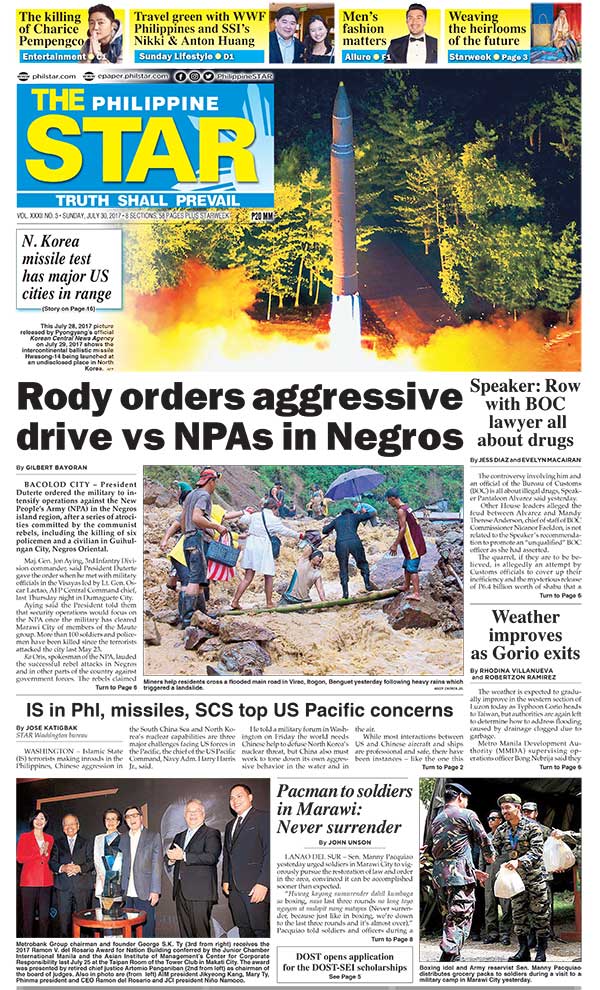**Detailed Caption:**

The image appears to be a screen capture of a vibrant and busy newspaper page, filled with multiple graphics and varied headlines. At the top, a collection of yellow, blue, and black boxes featuring images of dark-haired individuals with Asian features are prominently displayed. 

The first visible headline reads "The Killing of Charlize Pepcon." Directly below, other headlines include: "Travel Green with WWF Philippines and SS1's Nikki Inanon-Hanning," "Men's Fashion Matters," and "Weaving the Heirlooms of the Future."

Centered near the top, the newspaper's masthead, "The Philippine Star," is designed with "The" and "Star" in gold, and "Philippine" in blue, framed by a blue box. Below this header, the motto "Truth Shall Prevail" is printed in white.

A striking image of a rocket launching, with vivid orange flames emanating from its base and green trees in the background, accompanies the headline, "North Korea Missile Test Has Major U.S. Cities in Range."

Beneath this, another headline declares, "Rodrigo Duterte Orders Aggressive Drive Versus NPA in Negros," and is accompanied by an image of people traversing a rocky or muddy outdoor terrain.

Further down are additional headlines: "Speaker Row with BOC Lawyer All About Drugs" with accompanying text, "Weather Improves as Gorio Exits" with a paragraph of text, and "Pacquiao to Soldiers in Marawi: 'Never Surrender'," alongside images of soldiers carrying bags.

Towards the bottom of the page, another headline reads, "ISIS and Philippine Missiles: SCS Top U.S. Pacific Concerns," next to an image of individuals in formal suits against a stark black backdrop with more explanatory black text following it.